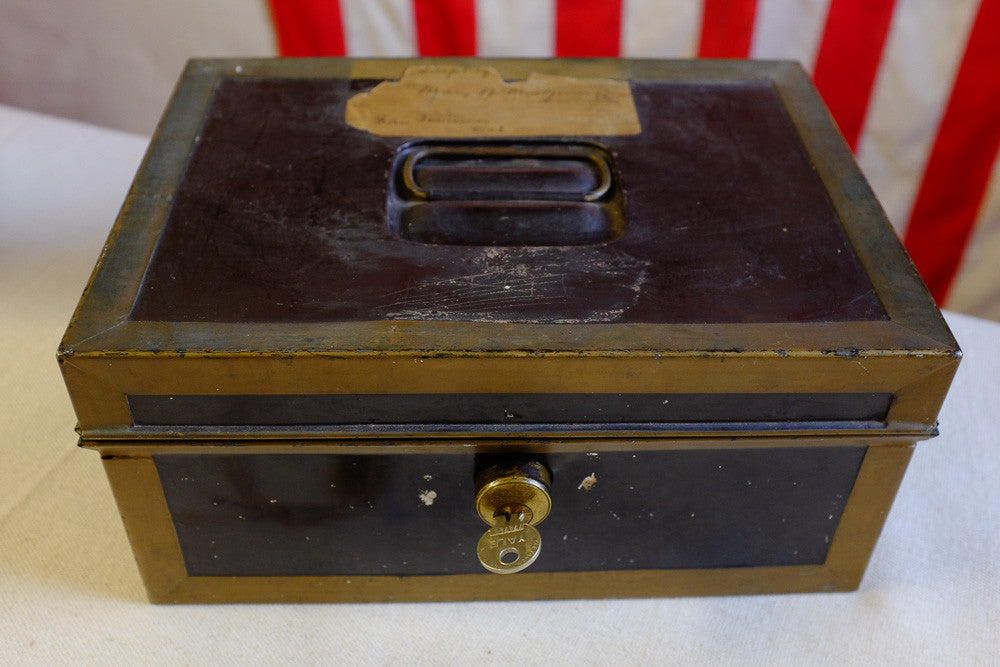An image depicts a well-worn, rectangular lock box with a gold trim along its edges and a predominantly black surface. The box, which is wider than it is tall, features a metal wire handle recessed into the top and a round, golden-bronze key inserted in the front lock. Scuff marks and speckles of rust and dust cover its surfaces, reflecting significant use over time. Affixed to the top is a faded, brown adhesive note, its text illegible due to wear and tear. The lock box sits on a white table, set against a blurred background where the red and white stripes of an American flag can be seen.